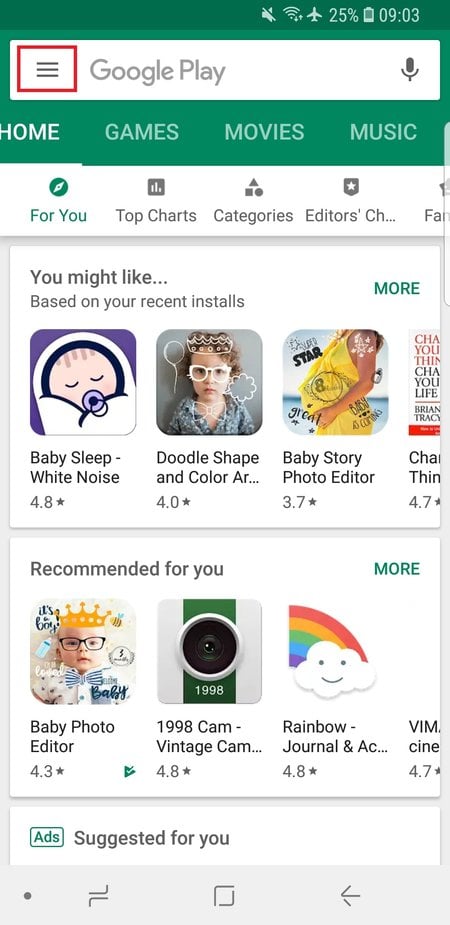A mobile phone screenshot of the Google Play Store interface. The phone’s battery level is at a concerning 25%, and the time displayed is 9:03. At the top of the screen, the search bar is labeled "Google Play." Just below the search bar are menu tabs: Home, Games, Movies, and Music, with the Home tab currently selected. Underneath these are submenus including For You, Top Charts, Categories, and Editor's Choice. The visible section of the Home tab displays a personalized section titled "You may like" based on recent installs, showcasing a list of apps such as "Baby Sleep - White Noise," "Doodle - Shape and Color," and "Baby Story Photo Editor," suggesting that the user may have a new baby. Further down, there's a "Recommended for you" section featuring apps like "Baby Photo Editor," "1998 Cam - Vintage," and "Rainbow Journal." The bottom part of the screen includes a "Suggested for you" section, which contains ads, but this part of the page is cut off in the screenshot.